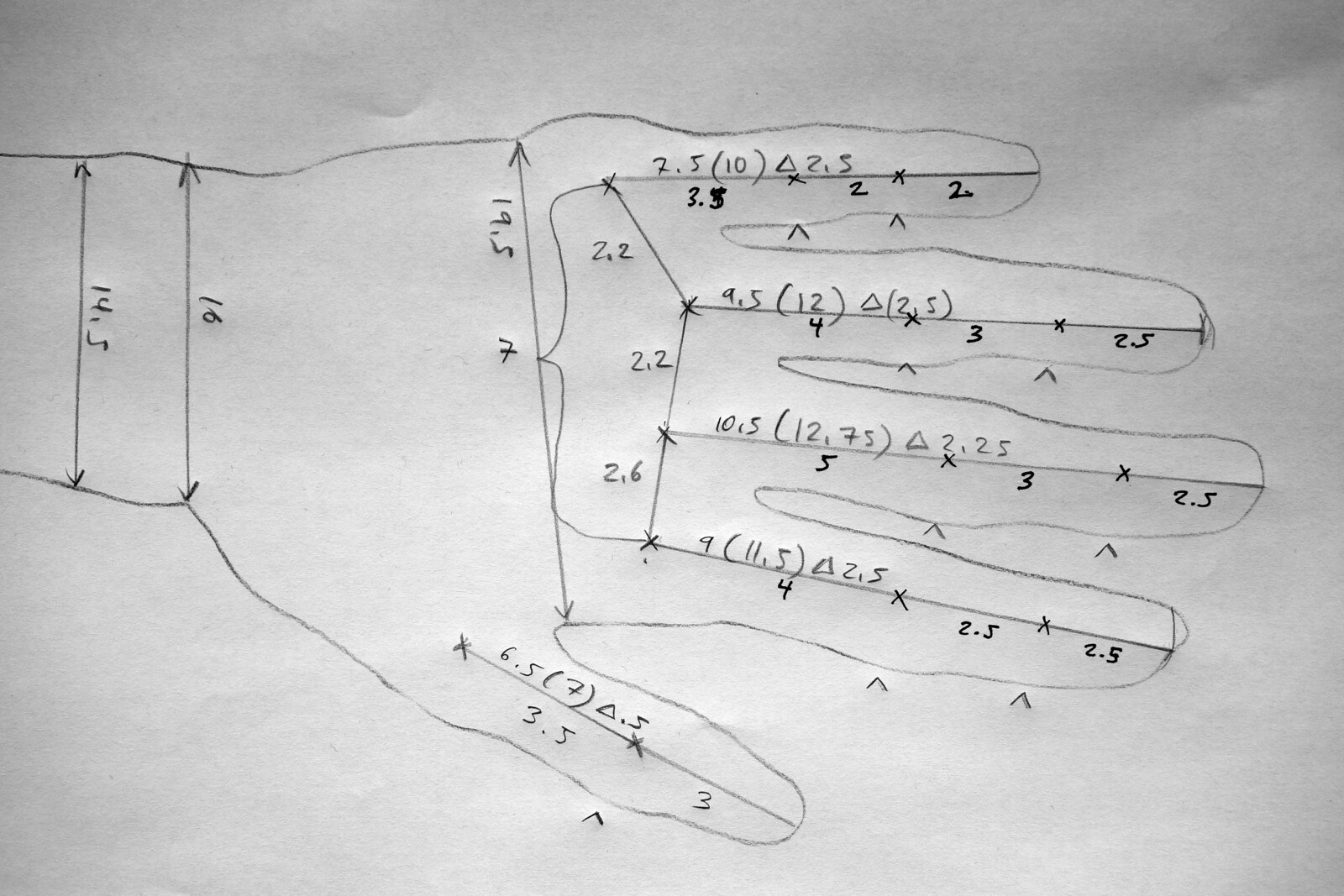This photograph features a piece of white printer paper that is notably wrinkled, particularly in the upper right corner. In the same corner, there's a visible shadow enhancing the perception of the wrinkles. The upper left corner has a distinguishable mark, likely made by someone on the reverse side of the paper, that appears to resemble the letter "C."

The main subject of the drawing is the outline of a left human hand, sketched in pencil with the pinky finger positioned at the top and the thumb at the bottom. Overlaid on this penciled outline, there are various lines and annotations made with a black pen. These annotations comprise a series of numbers and symbols.

Starting from the pinky at the top right, a line marks the beginning of these annotations and reads "2.5 (10) ▲ 2.5." Below this line, another annotation states "3.3 2 2." Moving to the next finger, there's a note of "4.5 (12) ▲ (2.5)." This pattern continues similarly across all the fingers, where each is marked with different numerical notations and symbols, providing a complex, detailed overlay on the penciled hand drawing.